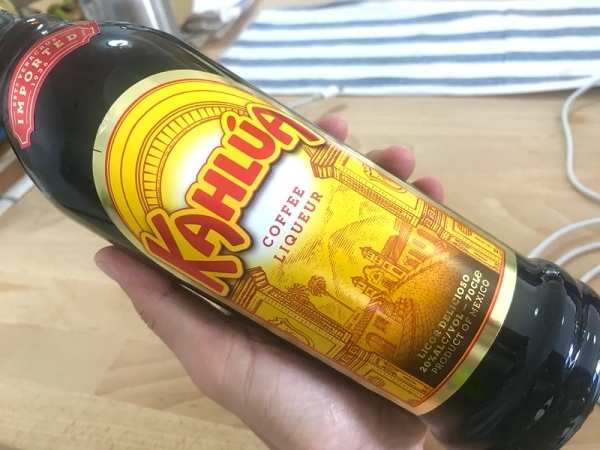In this image, the primary focus is a bottle of Kahlua coffee liqueur held in someone's hand. The bottle is positioned diagonally across the frame, extending from the top left to the bottom right. It is sleek and shiny, possibly plastic, with a prominent yellow label featuring the brand name "Kahlua" in bold red letters. Below the title, in smaller brown letters, it reads "coffee liqueur," and there is an intricate brown print design at the bottom of the label, depicting a house, road, and mountain. The bottle is described as containing 20% alcohol by volume and is marked as imported.

The scene is set inside a building, likely a house, with wood flooring covering most of the background. Additional items such as cords and objects scattered on the floor contribute to the indoor setting ambiance. The background also includes various colors: shades of gray, blue, yellow, red, orange, black, and different browns. Additionally, there is a blue and white rug partially visible near the top of the frame, juxtaposing against the tan-colored wooden floor. Overall, the image captures a well-centered, diagonally held bottle of Kahlua amidst a cozy, lived-in indoor environment.